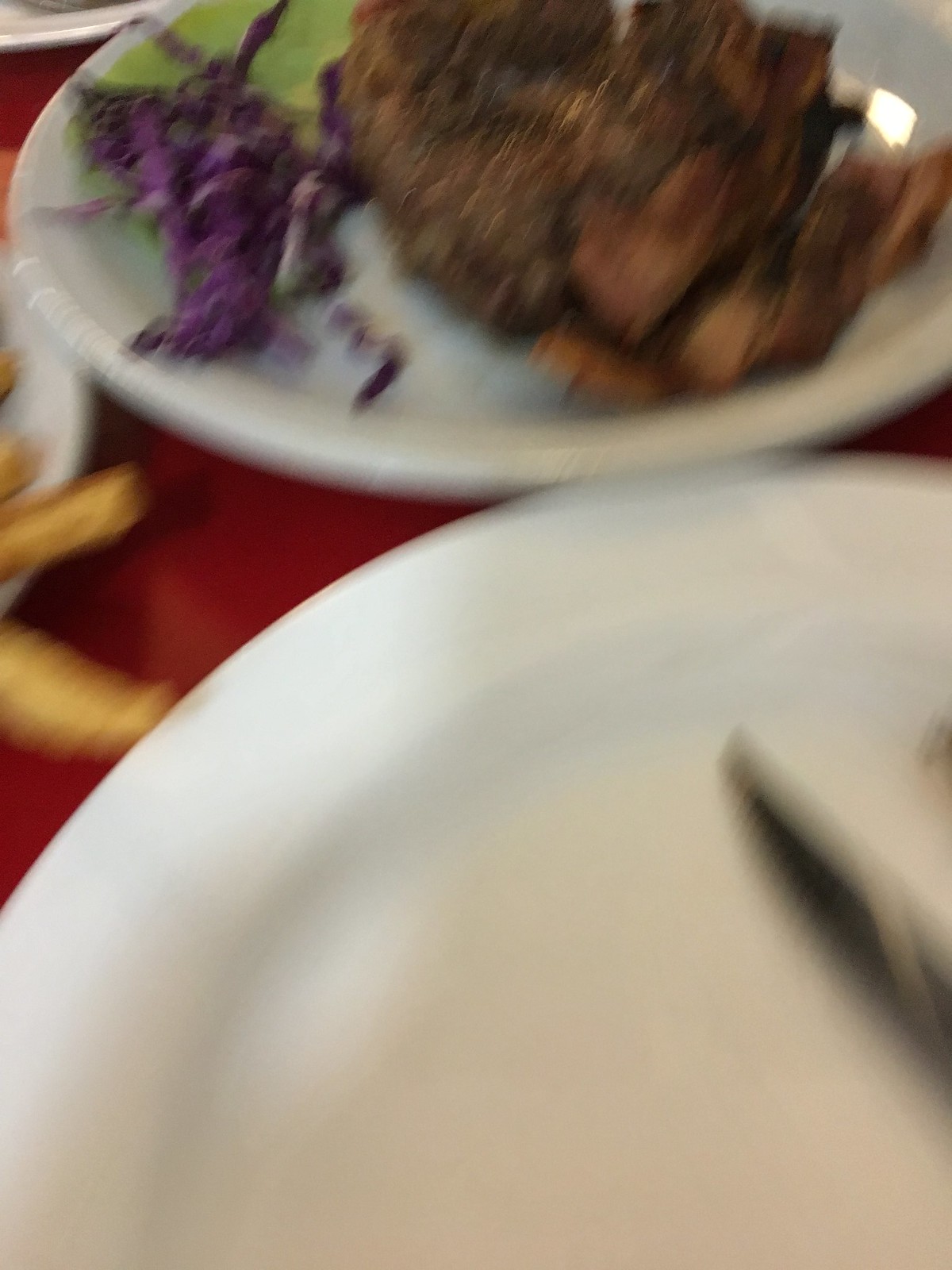In this slightly blurred color photograph, presented in portrait orientation, the foreground features a clean white plate adorned with a partially displayed silver knife. The enigmatic outline of another utensil—partially obscured—lies to the right of the knife. This setting rests upon a striking red tablecloth that extends beyond the plate. 

Dominating the upper portion of the image is another large white plate, prominently displaying a succulent beef roast from which a sizable section has been carved away. Nestled next to the roast is a portion of vibrant purple cabbage, finely chopped and adding a splash of color to the scene. Behind the beef and cabbage, a green leaf adds a touch of freshness.

Scattered across the table are additional white plates; one is almost completely out of frame in the top left-hand corner, and another plate laden with golden french fries is positioned just below the plate of roast, contributing to the inviting and abundant feast laid out on the red tablecloth.